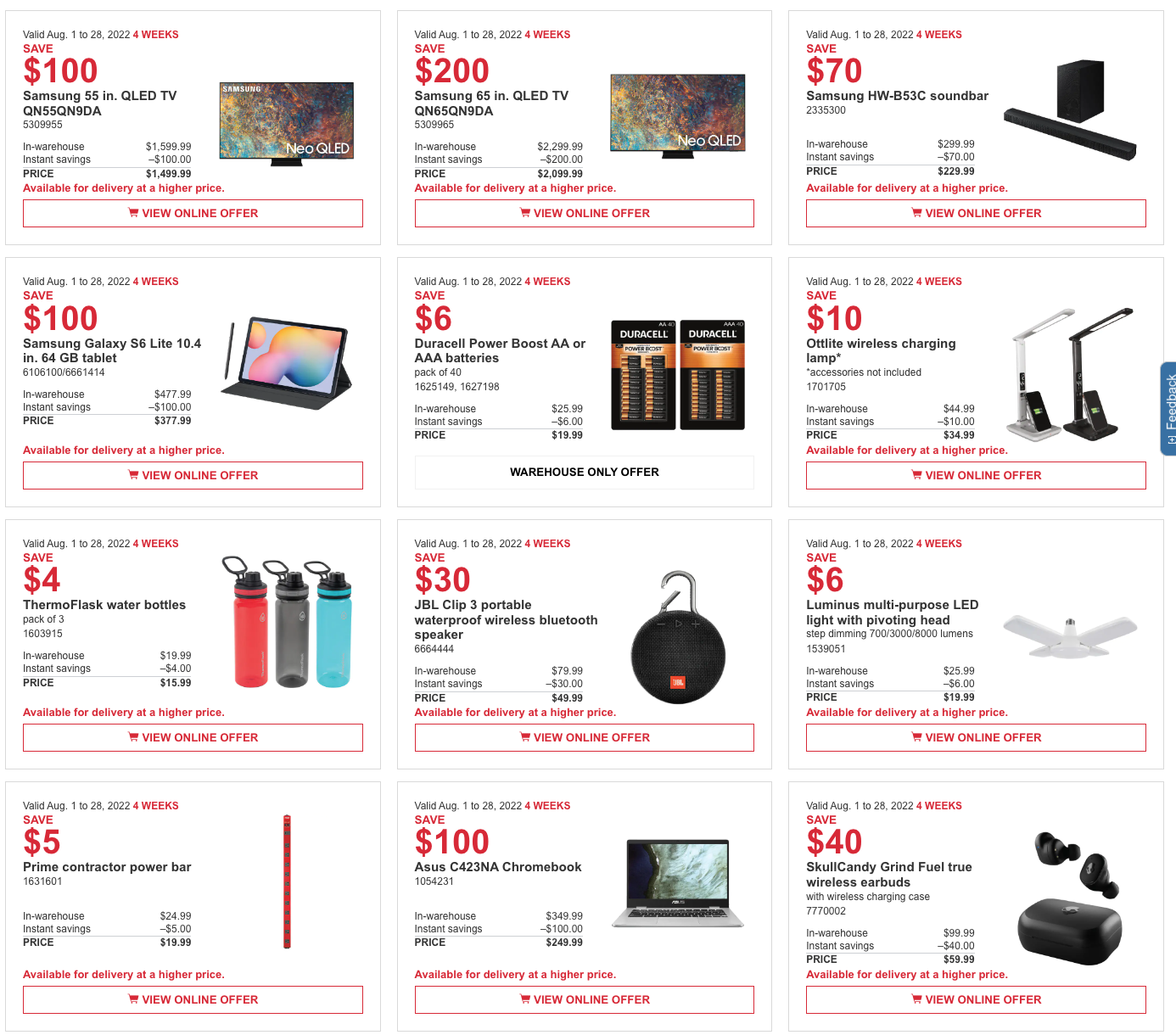The image depicts a detailed layout of a shopping website, showcasing various electronic and household products available for purchase. At the top of the page, there are two Samsung TVs displayed side by side, followed by a Samsung soundbar. Directly below these items, there is a Samsung Galaxy Tab S6 Lite 10.4 tablet. Next to the tablet, there is a pack of Duracell Power Boost batteries, available in both AA and AAA sizes. Adjacent to the batteries, there's an Off Light wireless charging lamp.

Moving to the third row of products, there are ThermoFlask water bottles, a waterproof wireless Bluetooth speaker, and a Luminous multi-purpose LED light with a pivoting head. At the bottom row of the display, you find a Prime Contractor power bar, an ASUS Chromebook, and a set of wireless earbuds.

Each product listing includes its price, a brief description, the validity period of the offer, and a clickable button to view the offer online. The overall layout is user-friendly, allowing shoppers to easily navigate and explore the available items.